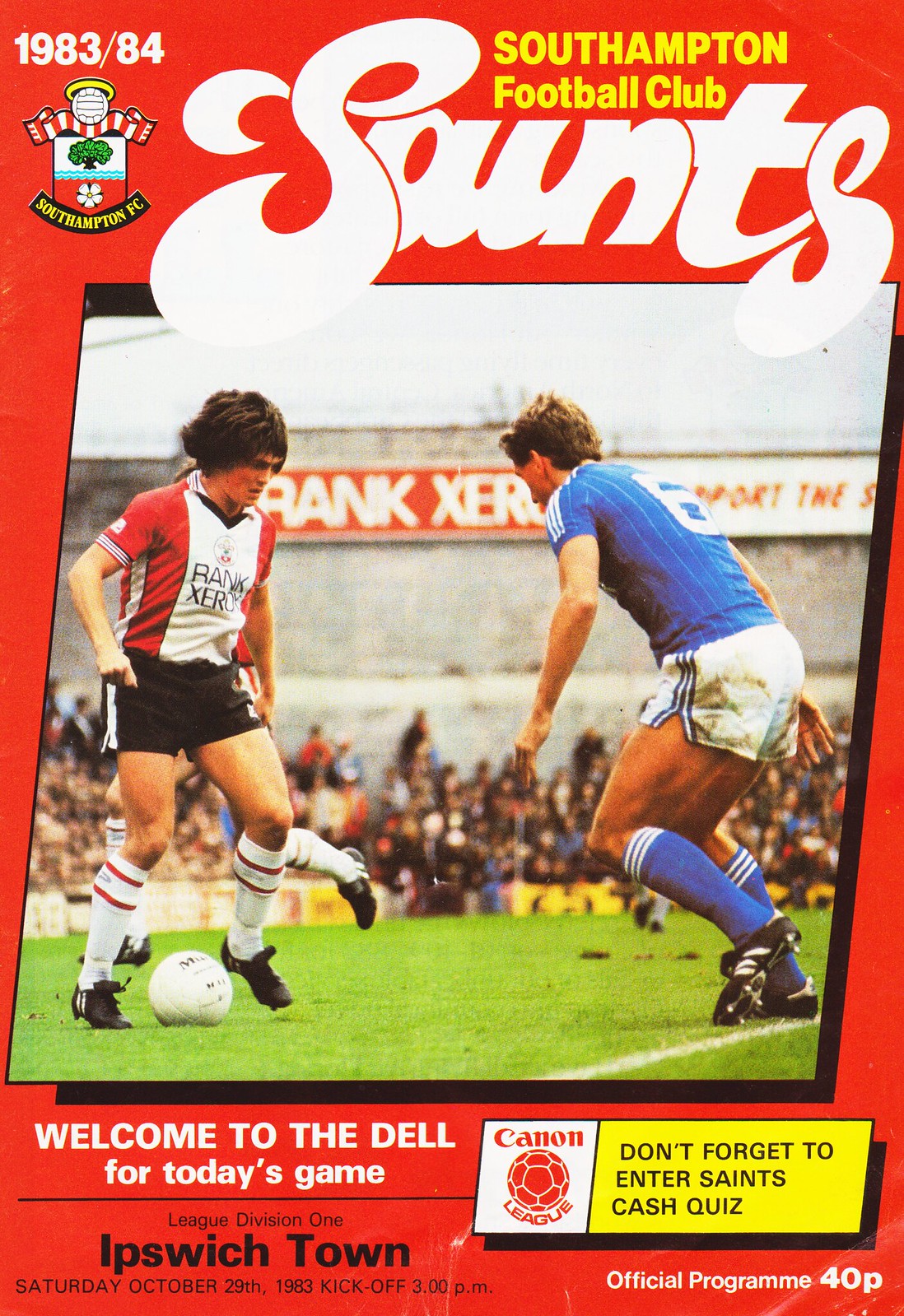This is an image of a vintage program for a Southampton Football Club game from the 1983-84 season. The cover is predominantly red with a striking white, bubbly title "Saints," and above it, in yellow letters, it says "Southampton Football Club." On the left, also in white, is the date "1983/84." The centerpiece is a vivid color photograph of two men engaged in a soccer match; one player is in a red and white jersey with black shorts, while the other is in a blue jersey with white shorts. A white soccer ball is situated between them on a green playing field, with spectators visible in the background. Towards the bottom, the text reads, "Welcome to the Dell for today's game: Ipswich Town," followed by "Canon League Division One - Saturday, October 29th, 1983, Kickoff 3 p.m." Additionally, in a yellow box, there's a reminder to "Don't forget to enter Saints Cash Quiz," and the program is noted to cost 40 pence.